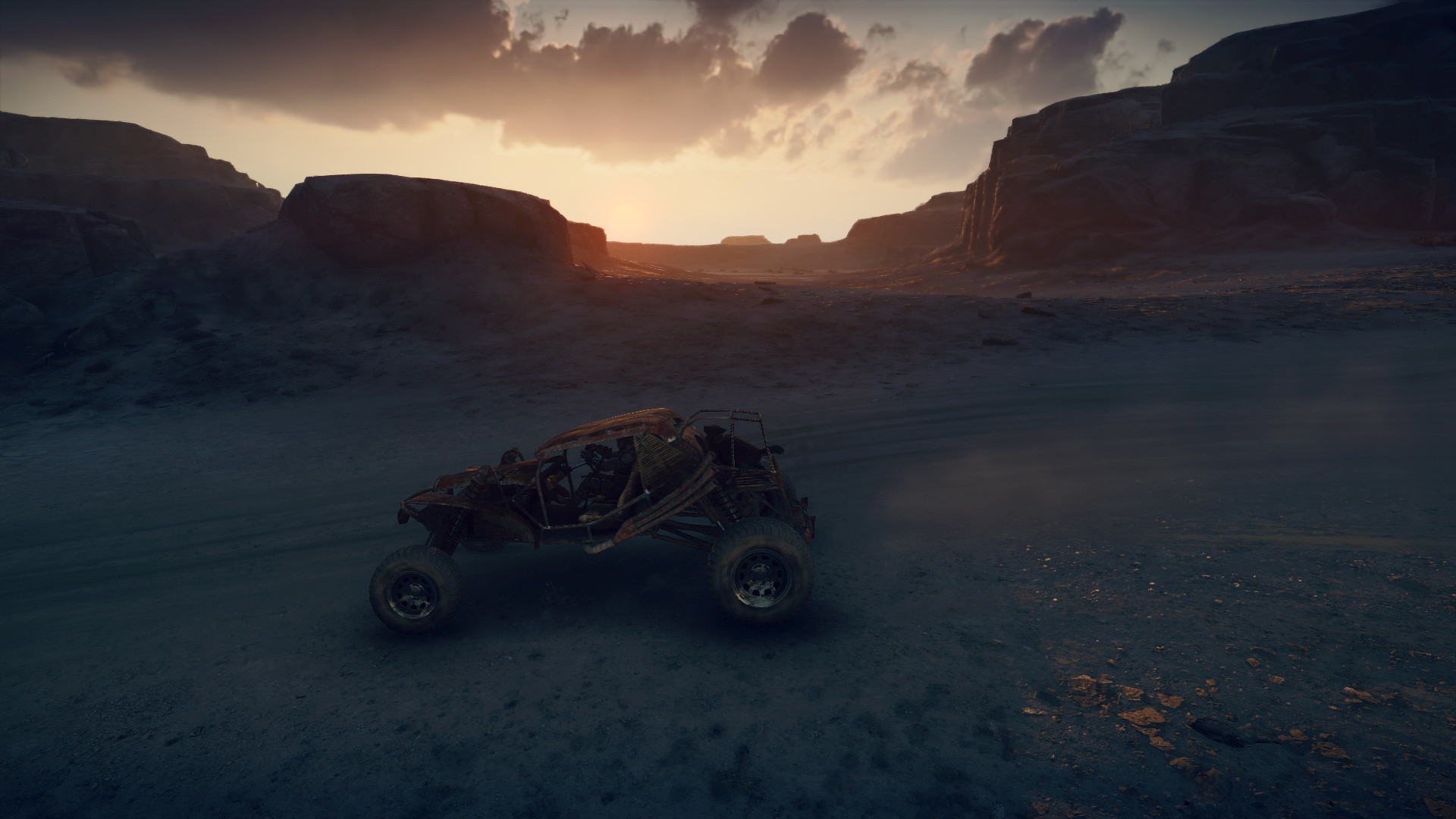In this striking image, we see an off-road vehicle situated in a desolate, gravel-strewn landscape under a setting sun. The vehicle, likely an ATV or dune buggy designed for rock crawling, stands prominently in the center of the frame. It's made from a tubular metal frame, largely uncovered except for a thin, rusted roof. With its robust, oversized rear tires and comparatively smaller front tires, this rugged machine looks somewhat incomplete, missing doors and other bodywork elements. The vehicle appears to be operated by a driver, visible holding the steering wheel. The dusty ground transitions into a curving gravel road, with the vehicle leaving a trail of dust behind. The backdrop features imposing, mountainous rocks with brownish clouds tinged by the setting sun's reddish rays, creating an atmospheric and almost eerie scene.